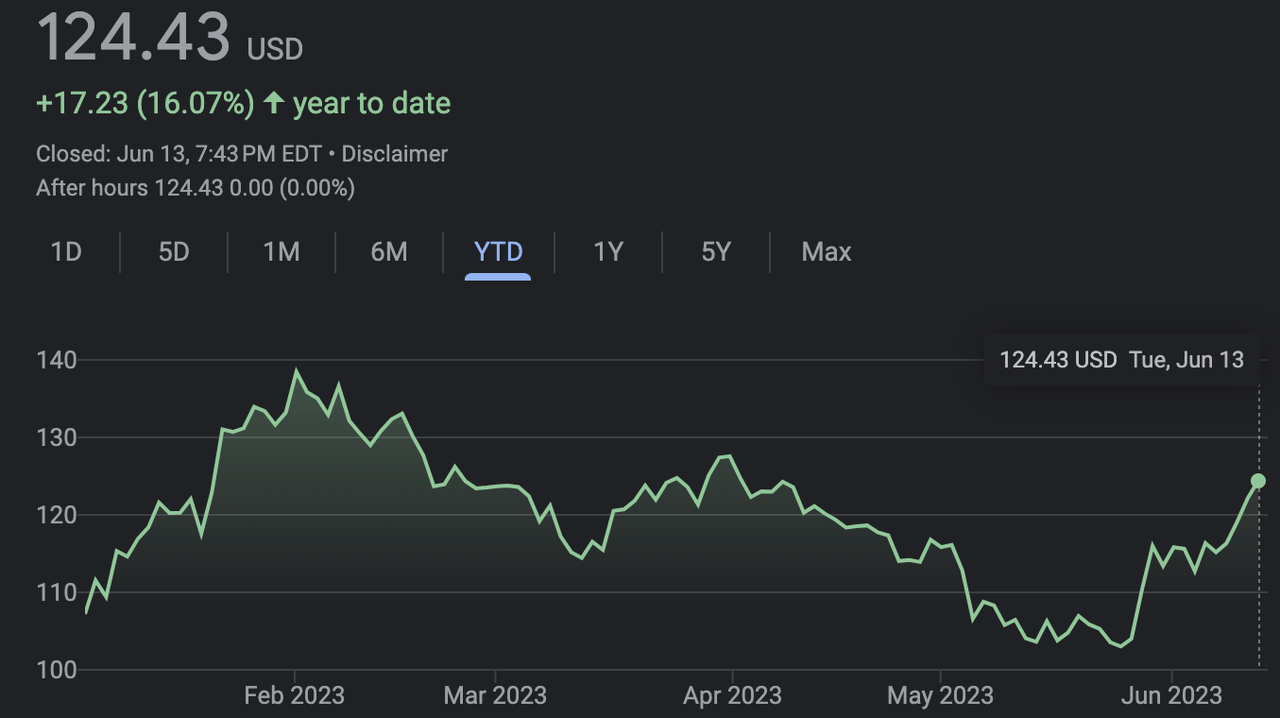The image showcases a desktop screen displaying stock trading software with a black background. In the center, the current stock value is prominently displayed in gray text as $124.43 USD. Below this value, in green text, the year's gain is shown as +17.23 (16.07%). Accompanying this is a timestamp in gray letters indicating the market closed on June 13th at 7:43 PM EDT, followed by a disclaimer. 

Under the main value, the after-hours trading value remains unchanged at $124.43, with no percentage change, both indicated by 0.00 and 0%. Just beneath this, a horizontal navigation bar lists various time intervals for stock performance: 1D, 5D, 1M, 6M, YTD (selected in blue), 1Y, 5Y, and max.

The graph itself depicts the stock's fluctuating value over time, with horizontal price markers at $140, $130, $120, $110, and $100. The timeline along the bottom spans from February 2023 to June 2023. The stock value line is jagged, illustrating volatility: starting around $110, peaking at $140, dipping to $115 in mid-March, rising to $130 in April, then falling to $105 in June before rebounding close to $125.